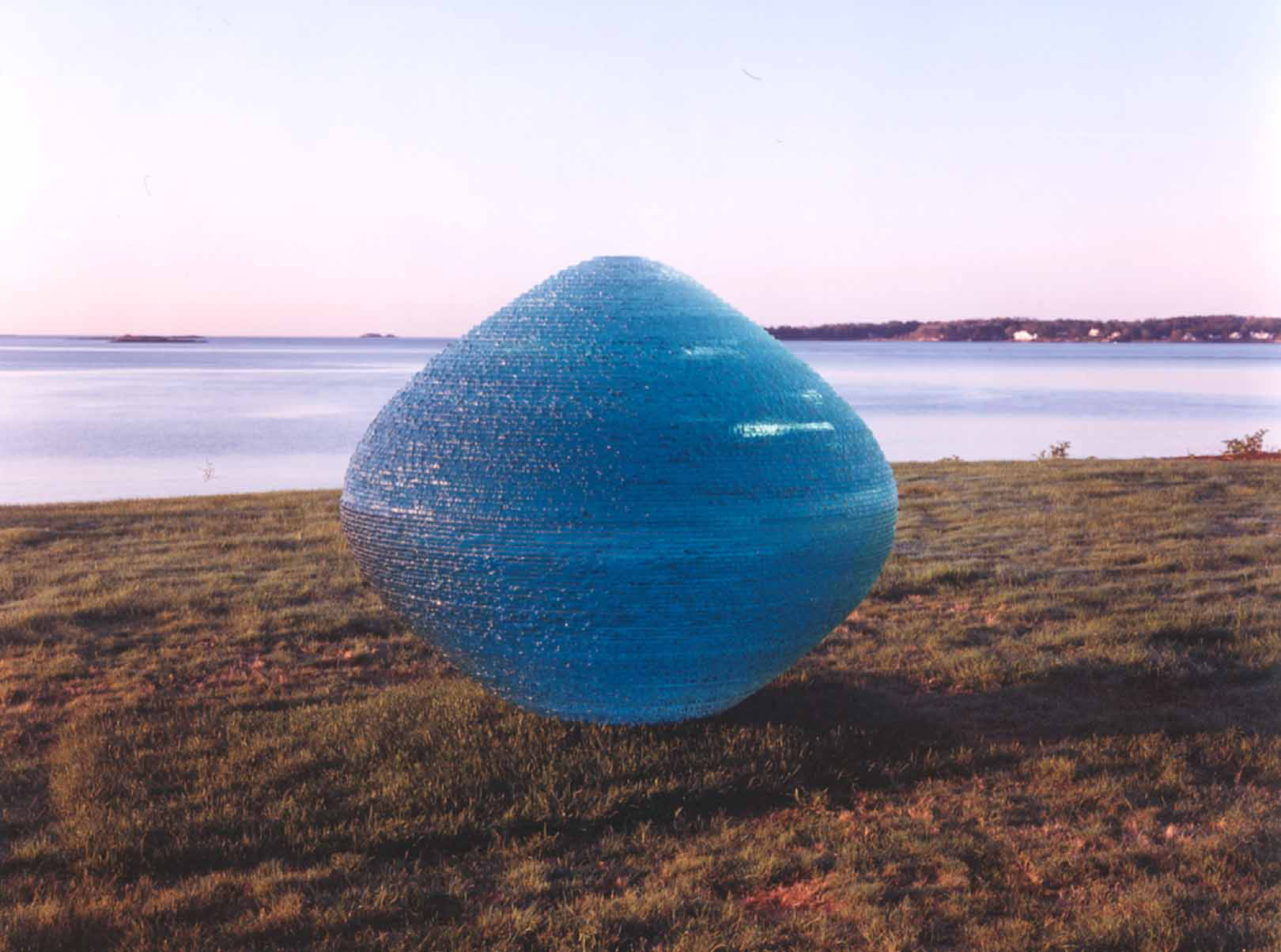The photograph captures a tranquil seaside landscape, characterized by a vast field of short grass in the foreground and a broad expanse of calm water stretching into the distance. The sky above is a soft bluish-gray, adding a serene backdrop to the scene. Beside the water, there are hills with scattered trees and houses, and these elements contribute to a peaceful, almost idyllic setting.

In the center of the image stands a striking glass art installation, its light blue hue beautifully complementing the surrounding landscape. The sculpture, resembling a rounded diamond shape with curved sides, is adorned with horizontal lines that segment it into layers, and textured dots or bumps that give it additional depth. The blue color of the sculpture transitions subtly between lighter and darker shades, with the middle section being the widest before tapering off towards the top and bottom. The entire scene, possibly captured during sunset, has a purplish tint that bathes both the landscape and the sculpture in a soft, warm glow, enhancing the ethereal quality of the composition.